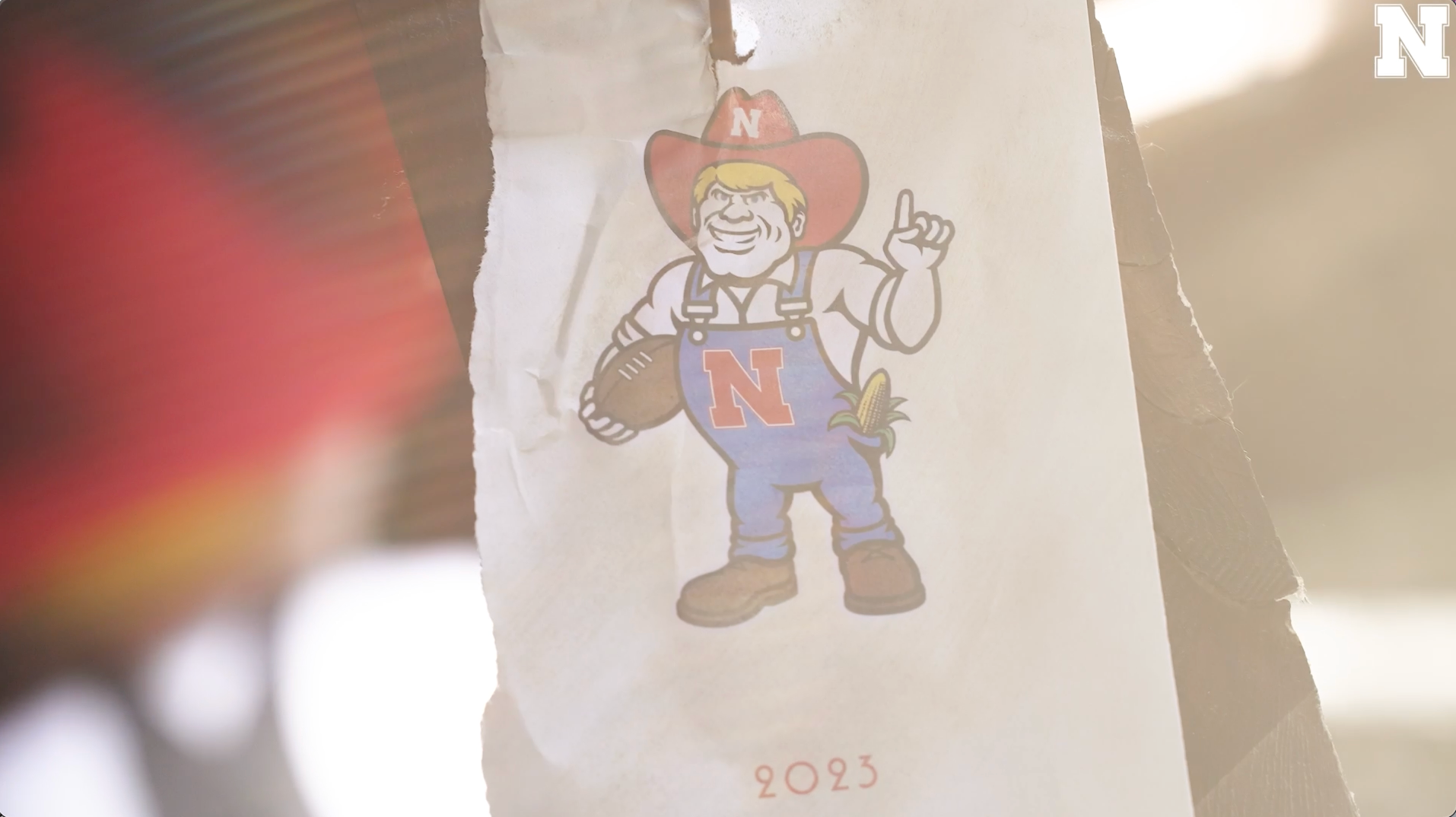This is a detailed close-up photograph of a sticker depicting the Nebraska Cornhuskers mascot. The sticker shows the jovial character, set against a piece of ripped white paper attached to a brown cardboard background, with a blurred section of red ribbed cardboard on the left. The mascot, instantly recognizable, features a large smile and short blonde hair topped by a red cowboy hat, marked with a white "N" in the center. He wears blue denim overalls that reach down to his brown boots, with a bold red "N" on the front. Underneath his overalls, he sports a white dress shirt, with his left sleeve pushed up to reveal a muscly arm holding a football. In his right front pocket, an ear of corn with a green husk sticks out. His right arm is bent at the elbow, and he proudly gestures with the number one finger up, signifying he's number one. This upbeat image of the mascot is clearly dated 2023, written in red beneath him.